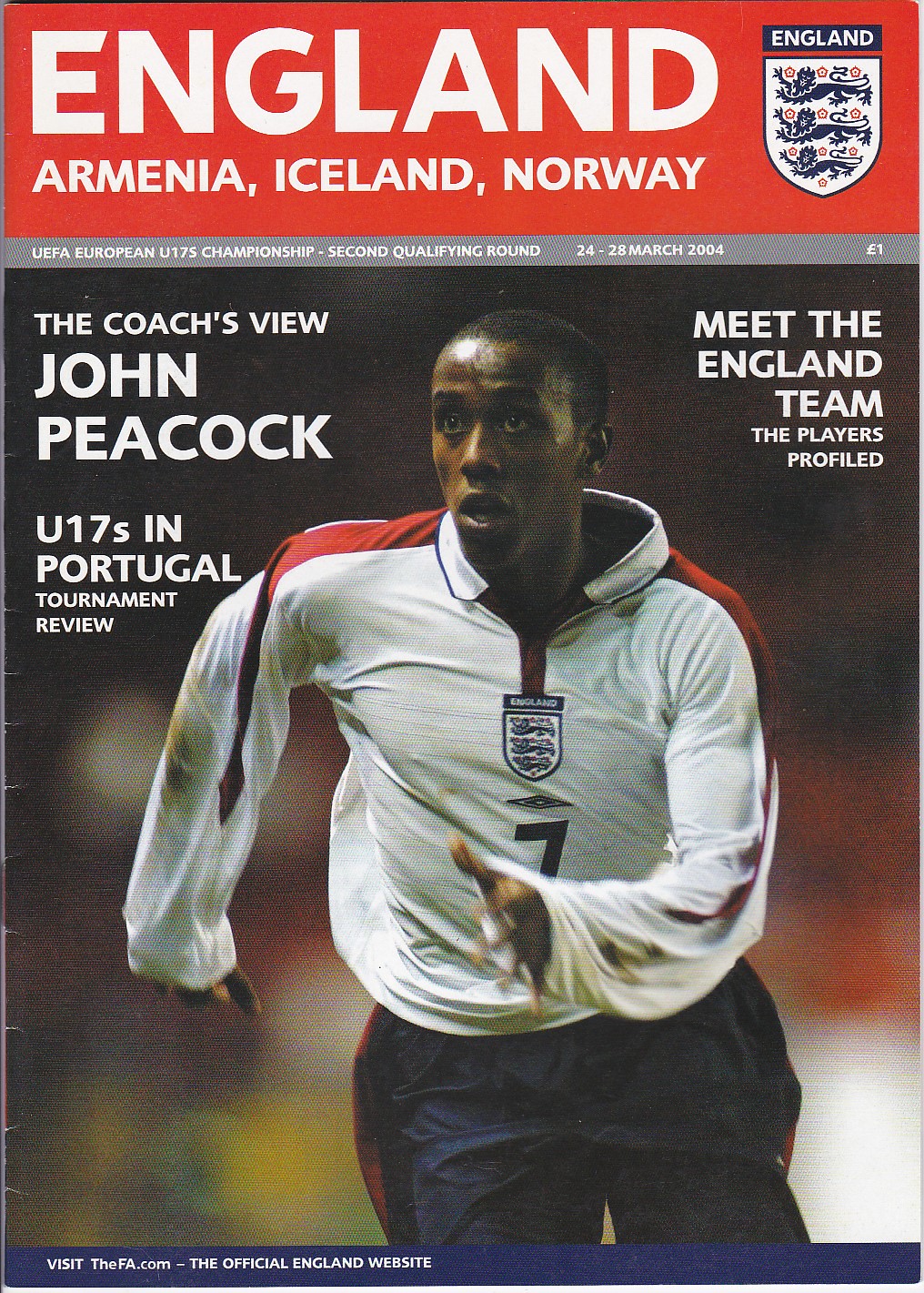The image displays a detailed cover of a game day program for a soccer event. At the top, a bold red bar features the text "England, Armenia, Iceland, Norway" in prominent white letters. To the right, there's the English coat of arms with three lions. Below the red bar is a grey section stating "UEFA European U-17 Championship Second Qualifying Round, 24 to 28 March 2004, 1 euro." Central to the cover is a large photograph of a black soccer player in motion, wearing an England jersey with the number 7. Surrounding the player, various texts provide insights such as "Meet the England Team, The Players Profiled," "The Coach's View, John Peacock," and "U-17s in Portugal Tournament Review."